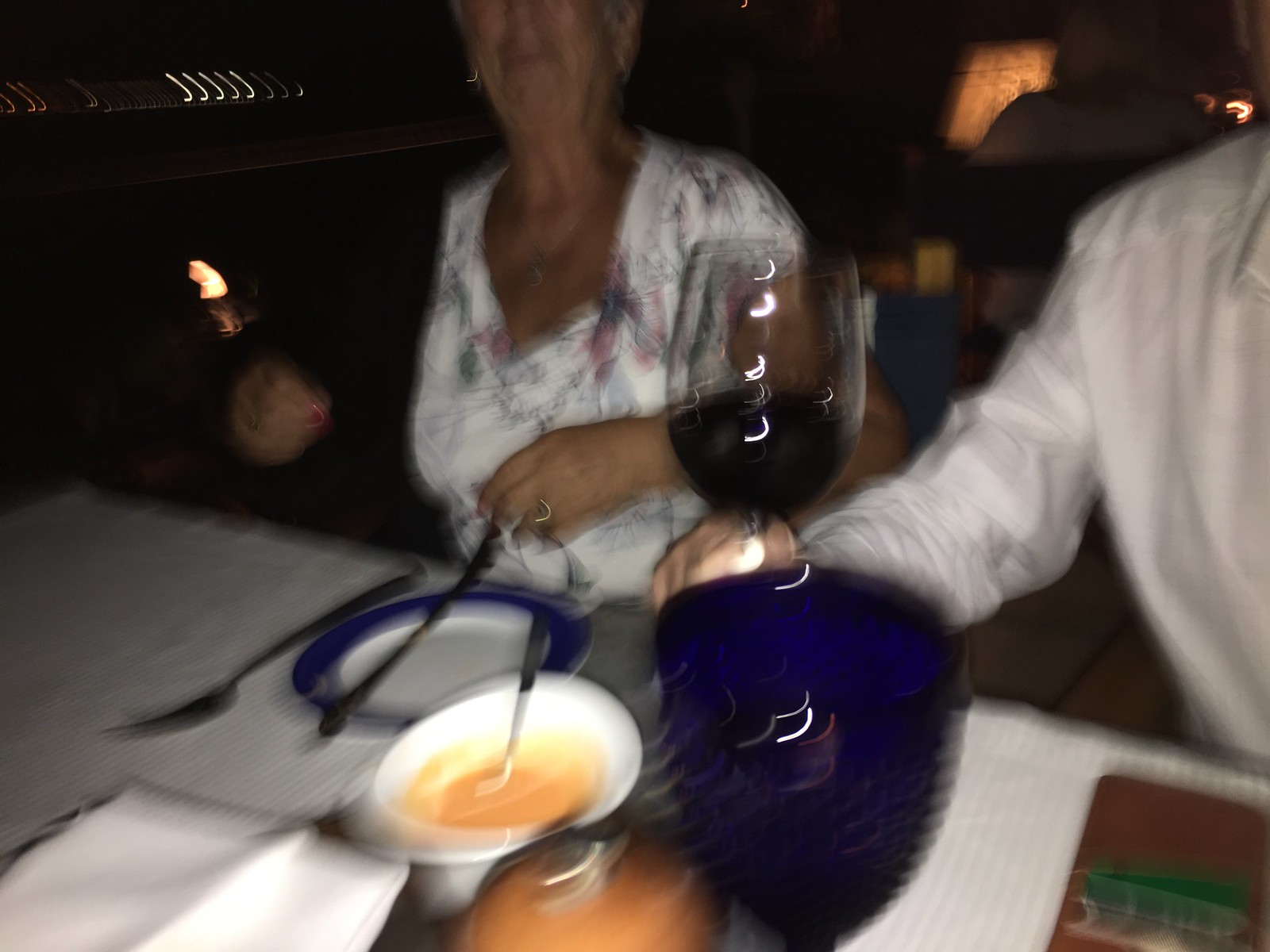In this blurry photo taken in a restaurant, a table covered with a white tablecloth dominates the lower section. On the left side of the table, there is an unidentified brown rectangle. At the forefront stands a striking cobalt blue goblet with a stem adorned with little round bumps on its body. To the left of this goblet is a white bowl containing a pale peach-colored sauce or liquid. 

In front of these items, there is a covered dish with a lid. The image also includes two indistinct figures. The person on the left is an older woman wearing a white top with floral patterns and a V-neck. Her short hair appears slightly disheveled, and her wrinkles are faintly visible. She has a plate before her with a deep cobalt blue ring around its edge, accompanied by a long fork and another indistinguishable utensil.

To the woman's left is an individual, presumably a man, dressed in a long-sleeved, collared, button-down shirt. Only half of his shirt is visible, and his face is obscured. His right arm is raised, holding a clear goblet filled with wine, which reflects light in the form of small, backward C-shaped white lines. Similar white lines can be seen on the upper left side of the image, the source of which is unclear.